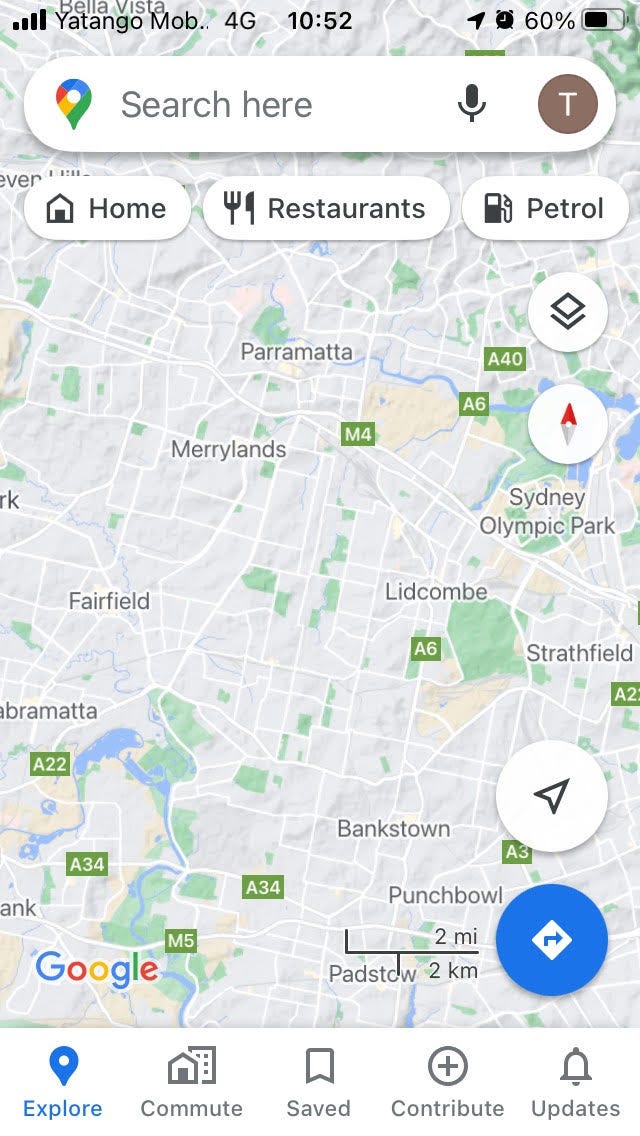**Detailed Image Caption:**

In this detailed screenshot of the Google Maps app displayed on a smartphone, we closely observe the interface and various elements that contribute to navigation and user interaction. At the very top of the screen, the status bar indicates full connectivity with four highlighted bars next to the text "Yetango Mob…," following which it truncates. Adjacent to this is the "4G" label, centered beneath the current time displayed as 10:52. To the right, the status bar shows four essential smartphone icons including an alarm symbol, a text reading "60%" indicative of user notifications, followed by a battery icon that shows the current level of battery charge.

Beneath the status bar lies a prominent white oval search bar bearing the text "Search here," prefaced by the Google Maps icon on the left and a microphone icon at its right end. Next to the microphone icon, a bold letter "T" encased within a dark circle is visible. Directly below this search bar are three quick-access search options: "Home" marked with a home icon, "Restaurants" denoted by a fork and knife icon, and "Petrol" signified by a petrol station icon.

The main map interface lies underneath these search options, displaying a colored map featuring various cities such as Maryland, Parramatta, Lidcombe, Sydney Olympic Park, Strathfield, Bankstown, Punchbowl, Fairfield, and Bella Vista. This map vividly illustrates street layouts and topographical elements along with the “Google” watermark positioned in the lower left-hand corner.

Flanking the right side of the screen are four vertically stacked circular icons serving navigational purposes. The bottom-most of these icons is highlighted in blue, showcasing a diamond white square icon with an arrow inside it, signifying a selected navigation function.

Along the very bottom are five tabs for different functionalities within the Google Maps app. The currently selected tab, "Explore," is displayed in blue, while the other tabs - "Commute," "Save," "Contribute," and "Update" - are available but grayed out, indicating they are not currently active.